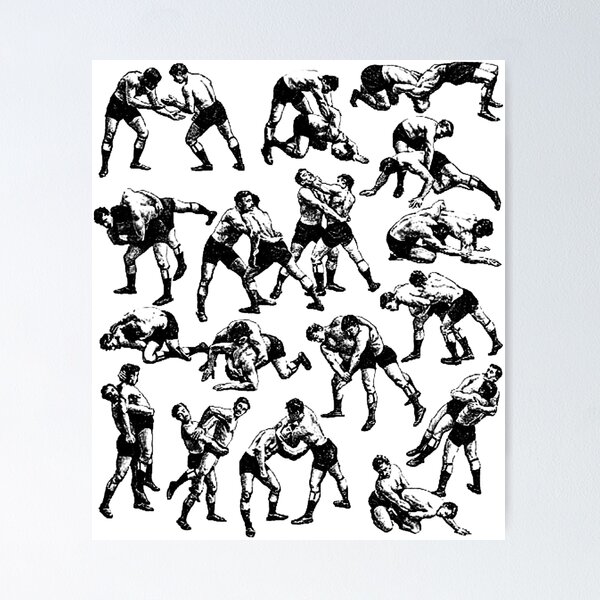The image is an old-fashioned black and white illustration depicting a detailed array of wrestling techniques and poses. The scene features two men, both wearing shorts, long socks, and shoes, engaging in various wrestling stances and moves. The men are depicted in 17 different positions, showcasing an assortment of holds, submission moves, and grappling pins. Notably, the top right-hand corner highlights an impressive suplex, where one wrestler is mid-air, his back arched towards the ground and chest facing up, while gripping his opponent's neck. This classic, advertisement-like drawing style resembles prints found on Trader Joe's bags, designed to offer viewers an overview of wrestling techniques, likely intended for instructional display in a gym setting.